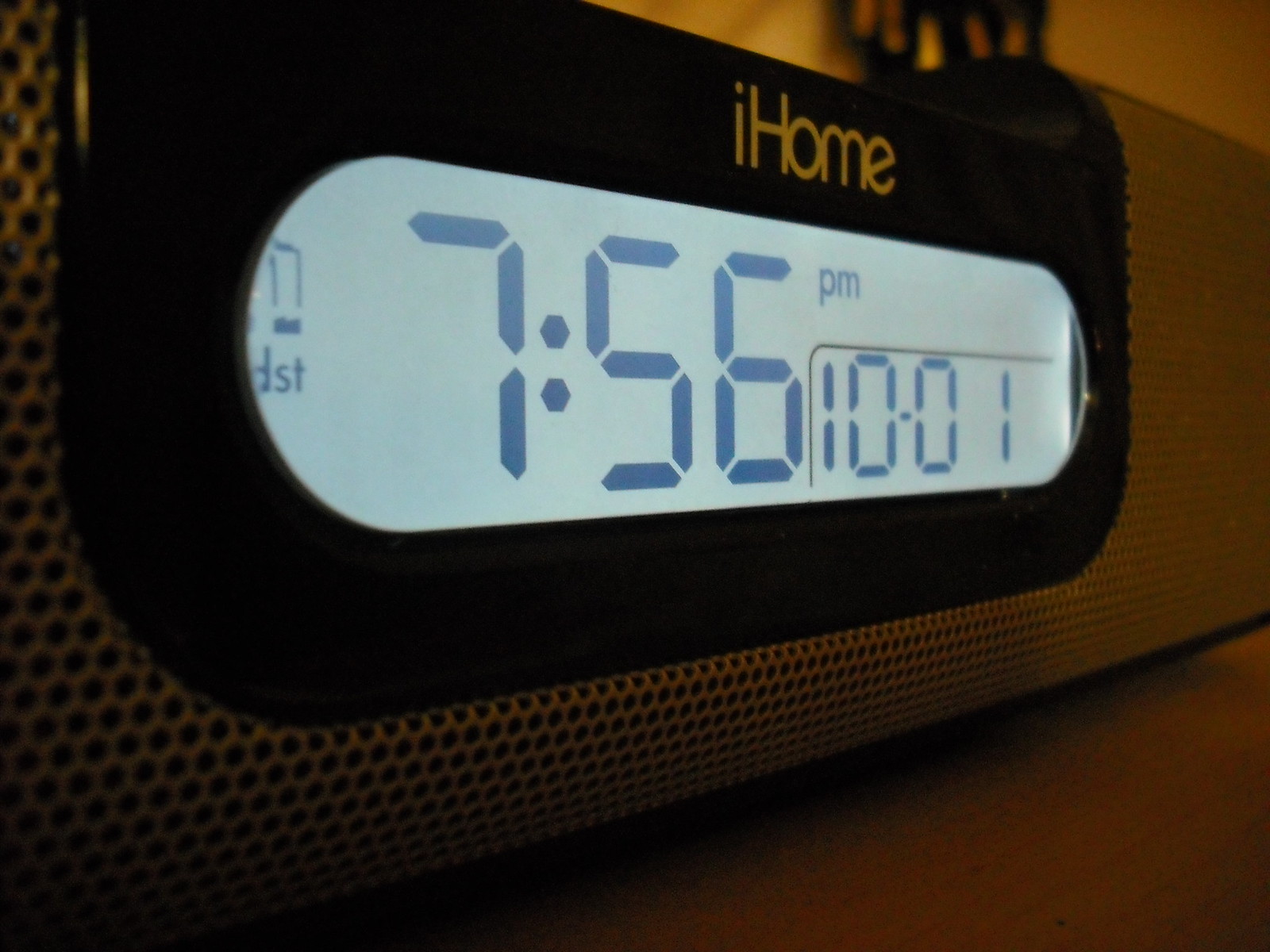The image displays an iPhone, prominently shown at the top against a backdrop that appears to be a grainy display screen. On the top left corner, some text is faintly visible, while the middle of the screen clearly shows the time as "7:56 PM." To the far right, the text reads "10-01." Attached to or projected on the display is a black square indicating an alarm. The speaker's grill plate is intricately patterned with numerous small silver holes, through which a black interior is visible. The surface beneath the iPhone is a wooden countertop with some black elements scattered around. In the upper part of the image and towards the back right, there's a yellow hue, possibly lighting, accompanied by what appears to be black boards or black metal structures.